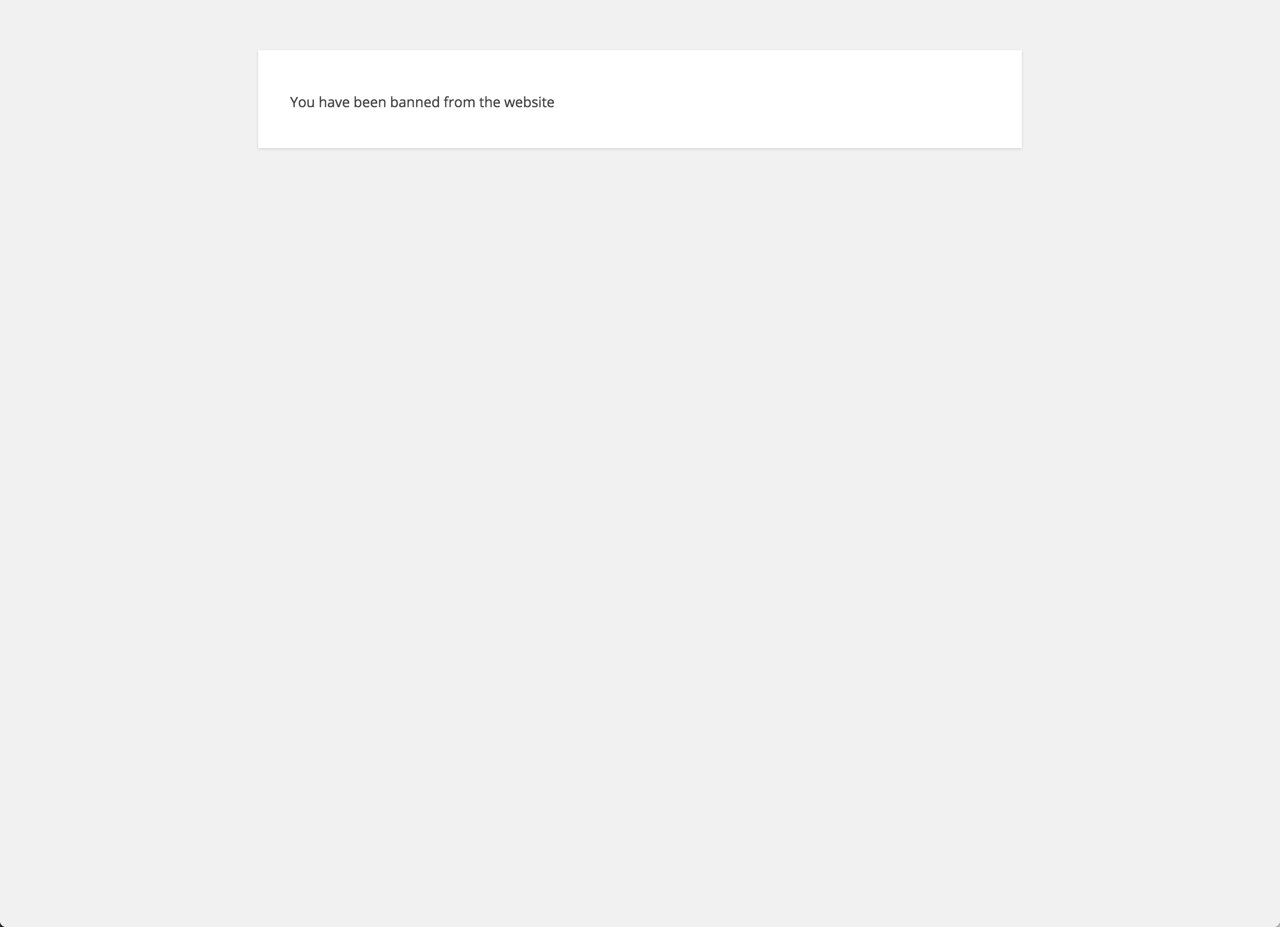The image consists of a light gray background. Positioned near the top, approximately half an inch from the top edge, is a small white rectangle that is horizontally centered. Inside this rectangle, on its left side, there is a line of black text that reads, "You have been banned from the website." The text is perfectly centered vertically within the rectangle, ensuring a balanced appearance. The overall design is minimalist and the message is clear and direct.